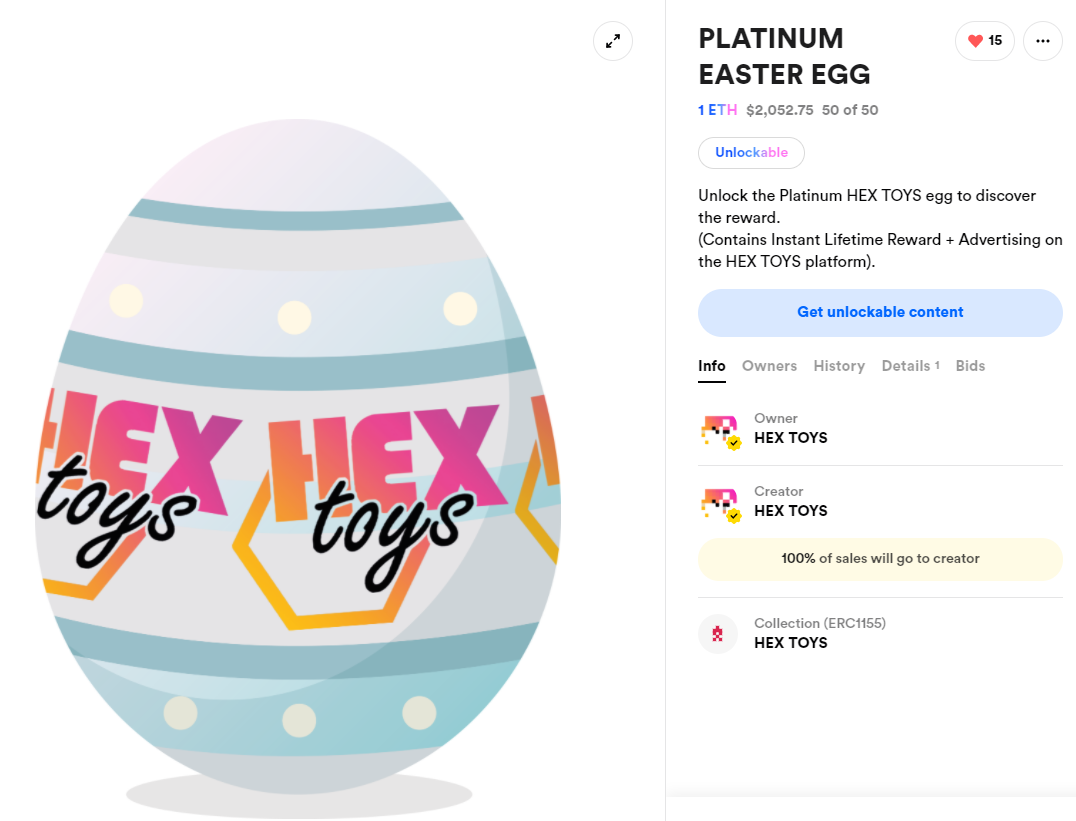The image is a screenshot featuring an Easter egg-themed illustration and accompanying details. The left side of the image showcases an intricately designed Easter egg with the text "Hex Toys" repeating around its center. On the right side, there is a detailed description of the item at the top, which reads: "Platinum Easter Egg 1ETH 2052 75 50 of 50." Below this, it states: "Unlockable: Unlock the Platinum Hex Toys egg to discover the reward. Contains instant lifetime reward plus advertising on the Hex Toys platform." A prominent blue button labeled "Get Unlockable Content" invites user interaction.

Below this section, various tabs are present, with the "Info" tab currently open. The visible information includes a list showing:
- Owner: Hex Toys
- Creator: Hex Toys

Additionally, a light yellow oval with black text indicates that "100% of sales will go to the creator." The final section provides details about the collection: "Collections (ERC 1155): Hex Toys."